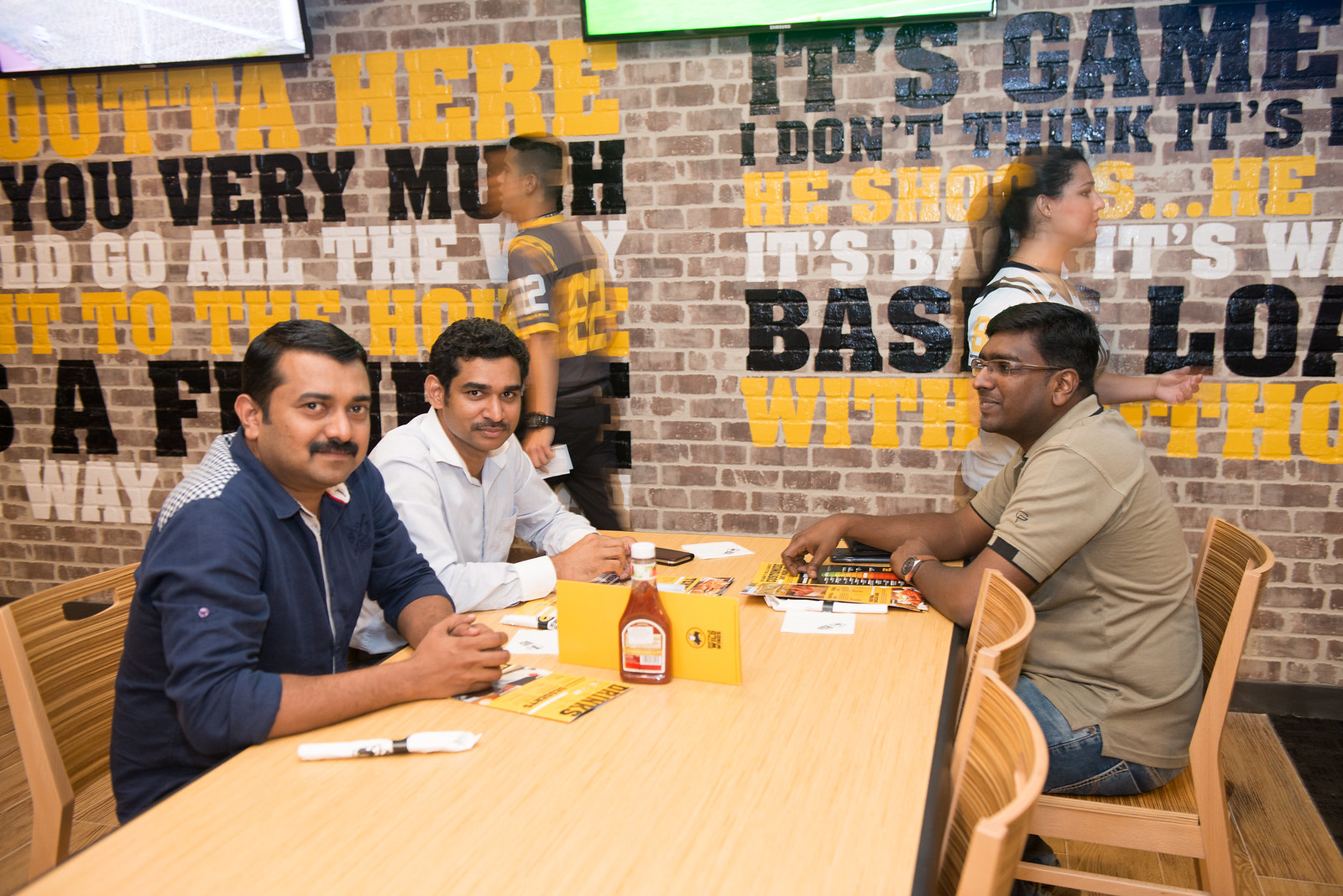In this color photograph, three men of Indian descent, likely in their 30s and 40s, are seated at a wooden table with matching wooden chairs in what appears to be an outdoor cafe or restaurant. The men have dark skin and hair; two of them sport mustaches. The man on the right is wearing a beige shirt and facing the left, smiling. Seated across from him, one man in the foreground is dressed in a dark blue zip-front jacket, while the man behind him wears a white shirt. The table is set with menus, cutlery, folded white napkins, and condiments, including a ketchup bottle.

Behind them stands a brick wall adorned with promotional lettering in bold yellow, black, and white colors. The text is partially obscured and reads phrases like "out of here, you very much" and references "games and events." Above the lettering, some TV screens are partially visible, cut off by the photo's frame.

In the background, a woman with a ponytail and a white shirt, possibly a waitress, walks to the right, while a man walks to the left, adding to the lively atmosphere of the scene. The image is in a landscape orientation, capturing a vibrant and bustling moment in this cafe or restaurant setting.